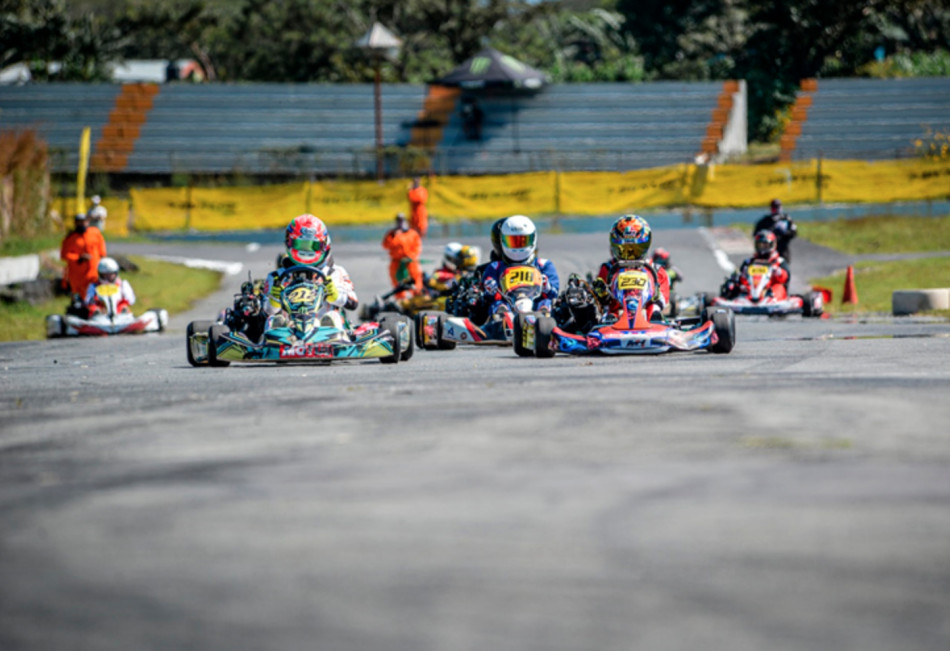The image captures an intense go-kart race with six to seven participants on a track, driving directly towards the camera. Three racers in the foreground are detailed prominently: the leader in a Spider-Man colored go-kart, followed by a racer in a Taco Bell Baja Blast colored go-kart, and a third racer in blue. The dynamic action is underscored by a blurred foreground due to the low-angle perspective. All the karts are vividly painted, and the drivers wear helmets with reflective visors, ensuring safety and a modern look. In the background, slightly out of focus, are three track marshals in brightly colored high-visibility suits, possibly mistaken for hazmat suits, ensuring the racers' safety. Behind them, blue bleacher seats with orange stairwell details are visible, mostly empty except for perhaps one spectator, shielded by canopied coverings. A chain-link fence in front of the bleachers is draped with yellow, black-lettered advertising, although it's too blurred to read. The scene is framed by patches of grass on either side of the track, grounding the setting in a typical outdoor race environment.